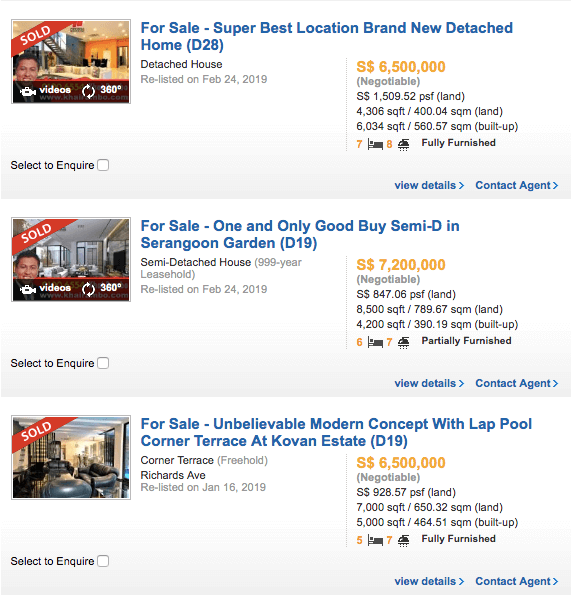Here is a detailed and cleaned-up caption for the given image description:

---

The webpage displays homes for sale, specifically showcasing new or detached homes. On the far left side, three photographs depict the available properties. The first listing features a detached house titled "For Sale: Super Best Location for Brand New Detached Home D28." This property, listed on February 24th, 2019, is priced at $6,500,000. It offers 4,308 square feet of living space on a lot measuring 1,508.52 square feet.

The second listing reads "For Sale: One and Only Goodbye Semi D in Sarangoon Garden." This semi-detached home carries a 999-year leasehold and was also listed on February 24th, 2019. With an asking price of $7,200,000, the property spans 8,500 square feet of living space on 847 square feet of land. A 999-year leasehold indicates that the ownership of the land is limited to a period totaling 999 years before it reverts and is resold thereafter.

The final listing advertises "For Sale: Unbelievable Modern Concept with Lap Pool Corner Terrace at Kovan Estate D19." This freehold property, meaning it can be owned indefinitely across generations, is priced at $6,500,000. The home offers 7,000 square feet of living space on a 928.57 square foot lot. Based on the characteristics of these listings, it appears that the properties might be located outside the United States, although the specific country is not mentioned.

---

This caption provides a comprehensive and structured description of the listings, highlighting key details such as property types, prices, land sizes, and lease terms.